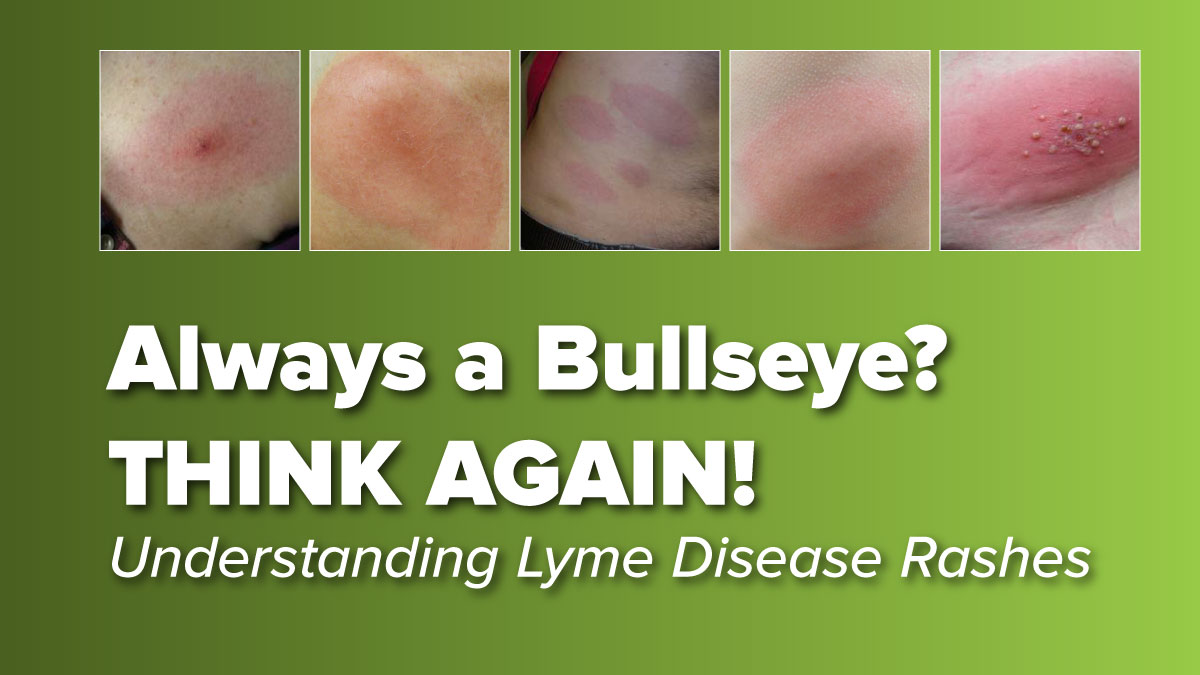The image is a green rectangle with a gradient that transitions from dark green on the left to light green on the right. The top third of the image features five white squares, each showcasing a different type of Lyme disease rash. The rashes vary: one square shows a single small red dot, another has a large reddish spot, the third displays multiple red spots, the fourth features a faint red spot, and the last square portrays a cluster of red bumps surrounded by a larger red area. Below these squares, large white text reads, "Always a bullseye? Think again." Additional smaller white text underneath states, "Understanding Lyme disease rashes," with the emphasis on providing a broader awareness of the diversity in Lyme disease presentations.